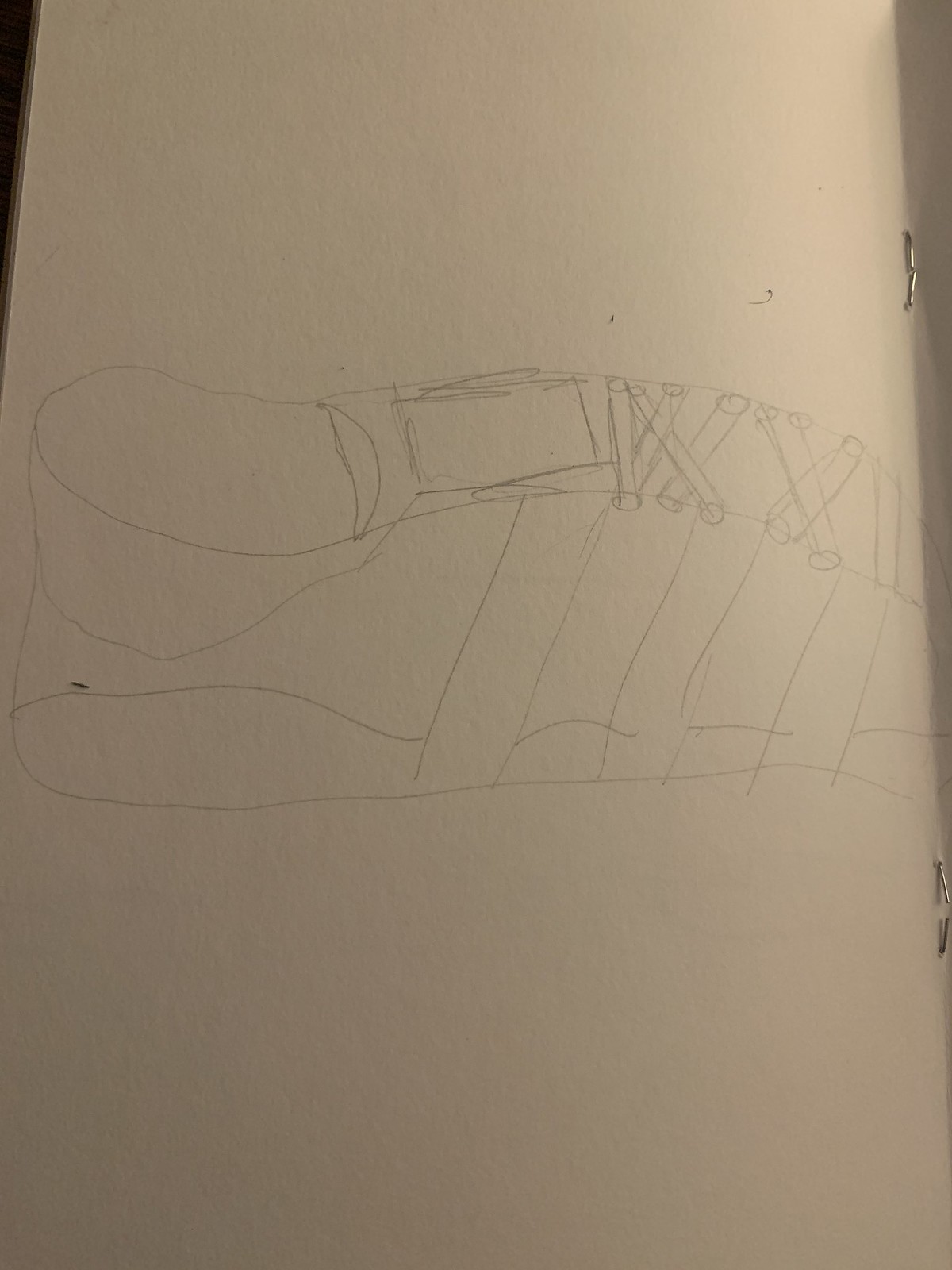In the image, we see a piece of white paper, possibly construction paper, featuring an abstract pencil drawing. On the top right, two tubes cross each other in an X-like formation. To the left of this, the drawing includes a squarish box that curves into a semicircle, tapering downward. Vertical lines are featured prominently, forming a pattern of small rectangles underneath. Near the left side, a curved line hooks underneath and extends across the page. Overlapping horizontal and vertical lines create an H-like shape below. The paper is stapled in the top and bottom right corners, suggesting it might be attached to other pieces of paper. The entire sketch is abstract, with various shapes such as oblong portions and conflicting geometries emphasizing its doodle-like nature.